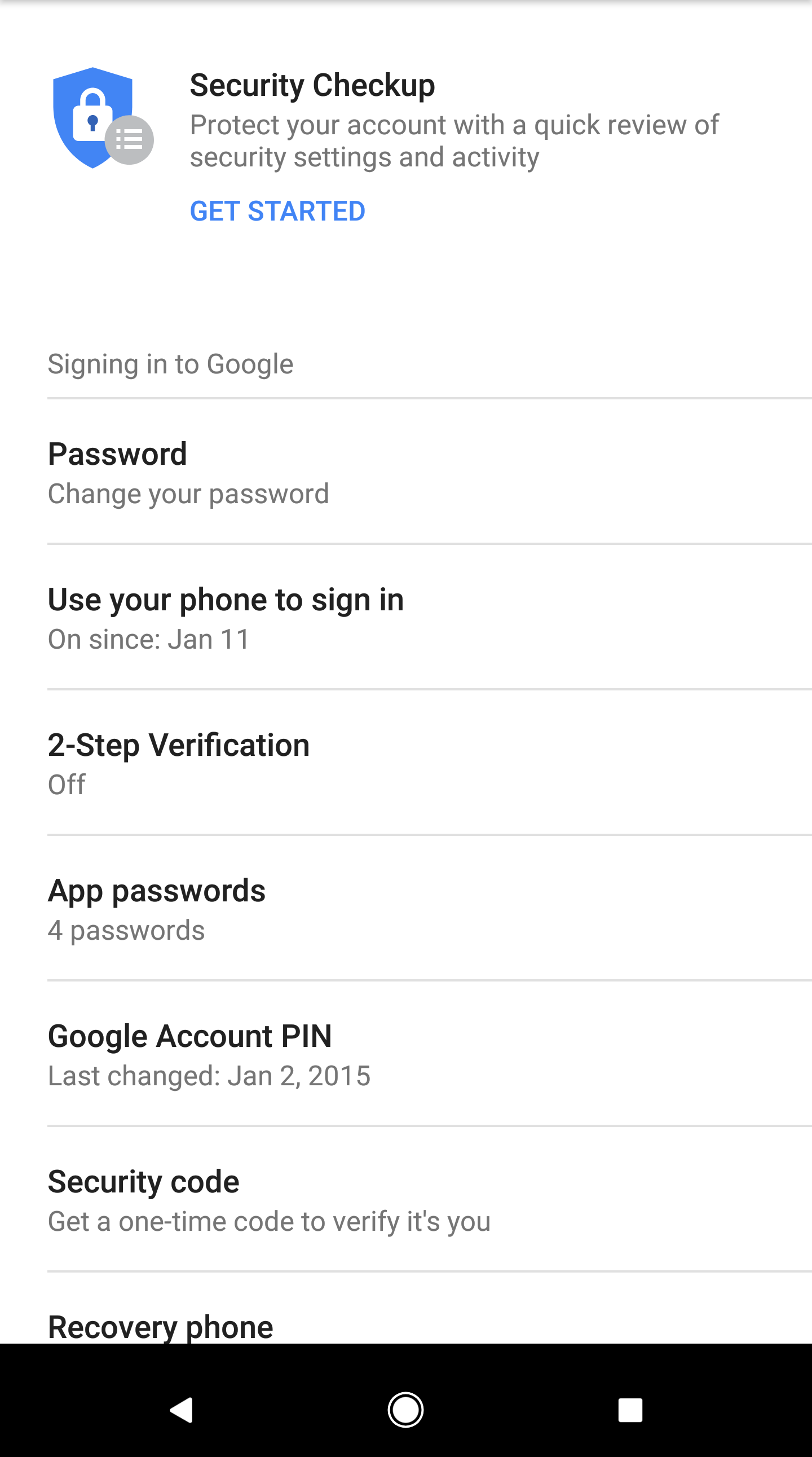**Detailed Caption:**

The image features a webpage titled "Security Checkup" at the top, prompting users to protect their accounts by reviewing their security settings and recent activities. The call-to-action text "Get started" is highlighted in blue. To the left, there is a blue shield icon with a white lock symbol, indicating security.

Below the main header, the content is structured in a list format with white bullet points. These bullet points detail various security settings and activities, including:
- "Signing into Google" with a note on password changes
- Instructions on using a phone for sign-in, noted as enabled since January 11th
- Information about two-step verification, which is currently off
- App passwords details
- Last change of Google account PIN was on January 2nd, 2015
- Option to get a one-time security code for account verification
- Recovery phone information, although it is partially cut off in this image

The entire text is left-justified, with lines separating each entry for better readability. The bottom of the page features a navigation bar with a backward arrow, a circular icon, and a square icon, all set against a black background. The text on the page predominantly uses black, white, and gray fonts, with blue used sparingly for emphasis, ensuring a clean and professional appearance.